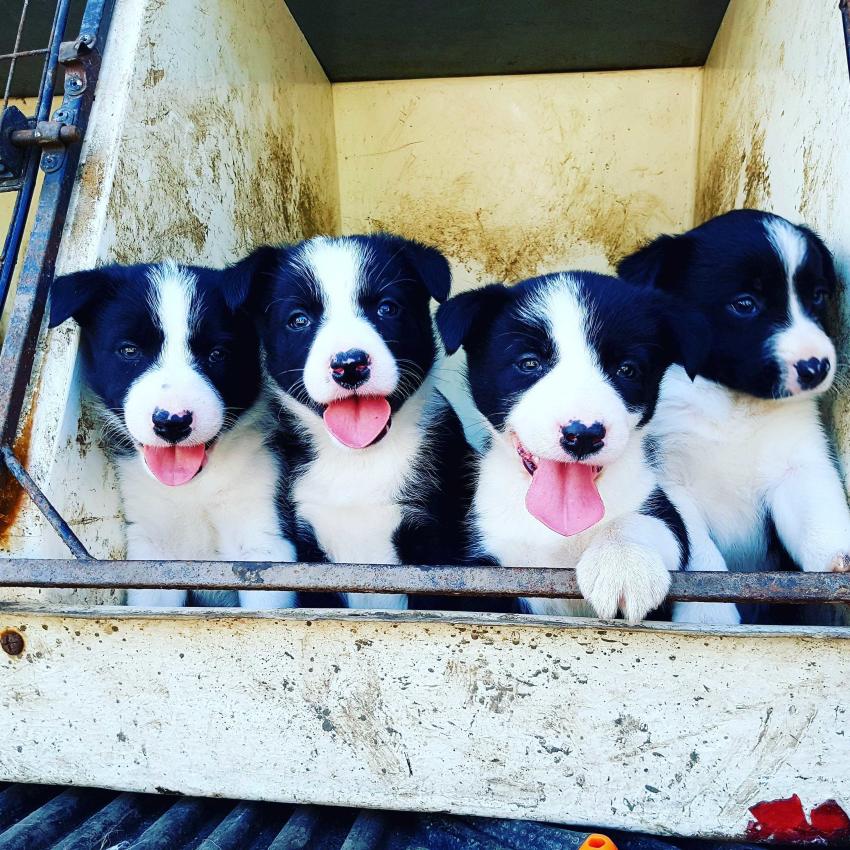This charming photograph features four black-and-white puppies nestled inside a somewhat dirty white plastic crate, which has visible brown splotches and a yellowish tint towards the top. The puppies share a striking resemblance, each displaying primarily black fur accented by white stripes that run down their faces to their white paws. Three of the puppies happily have their pink tongues hanging out, exuding an air of joyful playfulness. The fourth puppy, positioned to the right, stands out with its serious expression and mouth closed, casting a curious gaze to the side. The open crate reveals an intricate setting, with a black metal grate to the left and a silver handrail that one of the puppies leans against with its paw. The detail of their alertness and attentive stares into the camera adds to their captivating cuteness, making the scene immeasurably endearing and inviting.